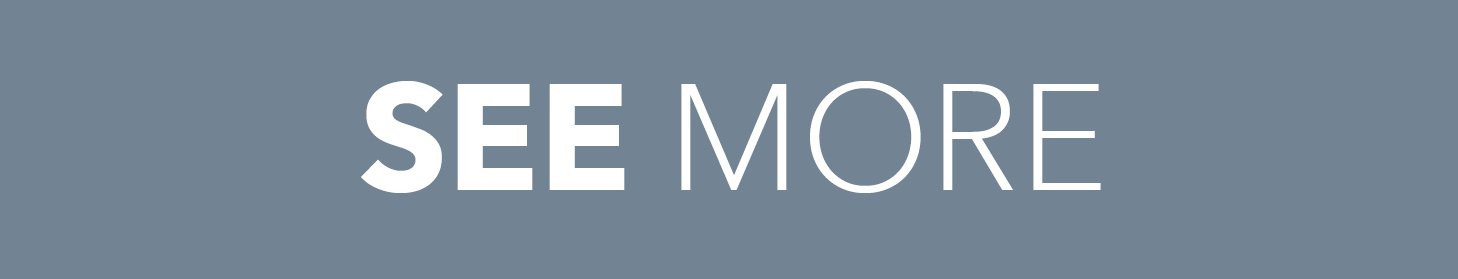The image is a horizontally-oriented, computer-generated graphic with a rectangular shape, approximately 6 inches long. Its background features a dark, gunmetal grey, bluish-green hue that is plain and without texture. Centrally aligned on the rectangle are two words in bold, white, all-capital letters: "SEYMOUR". The first part, "C", is depicted in large, block-style font, making it stand out. This is followed by "MORE", which is in a thinner but still block-style font, creating a contrast in thickness while maintaining uniformity in height. Notably, the letter "O" in "MORE" appears larger compared to the other letters. The overall design is simple and clean, with ample negative space around the text, creating a striking visual emphasis on the words.